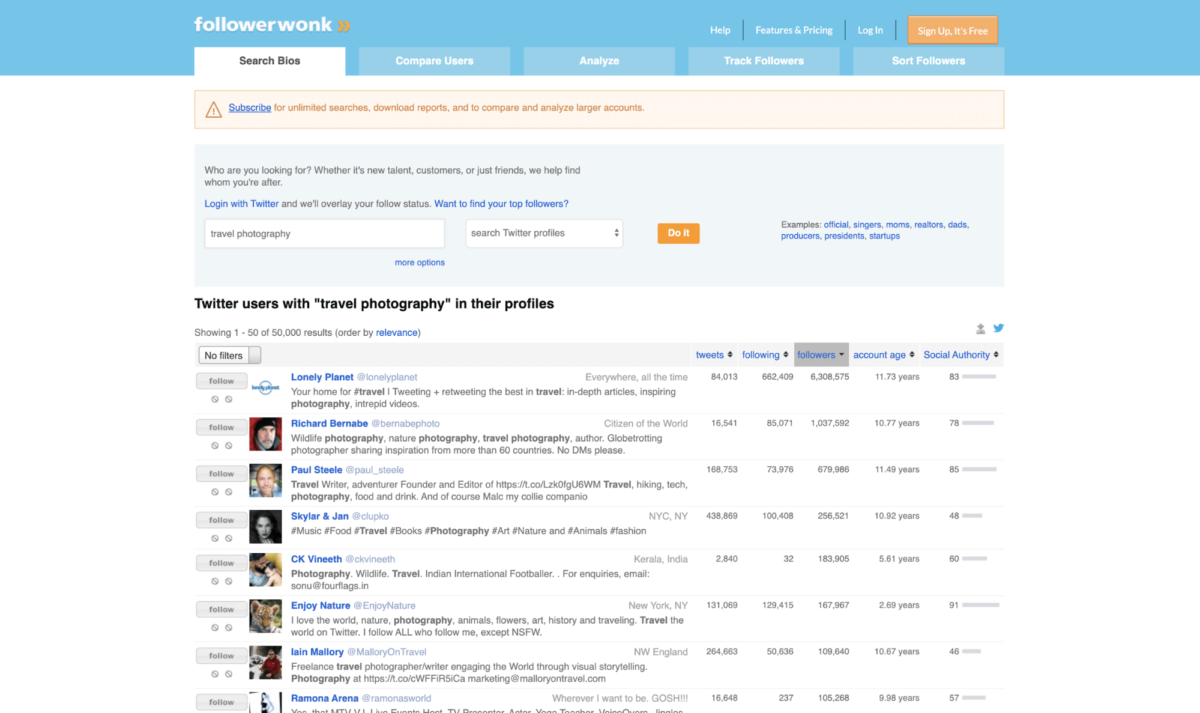This screenshot features the Follower Wonk website, which boasts a clean, aesthetically pleasing design in baby blue and white. At the top left, the website's name, "Follower Wonk," is displayed alongside twin right-facing yellow arrows, adding a distinctive touch to the branding.

Below the site name, the navigation bar includes several tabs: "Search Bios" (currently highlighted in white, indicating the active page), "Compare Users," "Analyze," "Track Followers," and "Sort Followers." Above this bar, the upper right corner offers additional options: "Help," "Features and Pricing," and "Login." Notably, there is an orange button labeled "Sign Up - it's free."

Directly beneath the navigation bar, a yellow caution message reads, "Subscribe" (underlined and hyperlinked in blue) followed by the benefits of subscribing: "For Unlimited Searches, Download Reports, and to Compare and Analyze Larger Accounts."

A gray information box situated beneath the caution message prompts users with, "Who are you looking for? Whether it's new talent, customers, or just friends, we help find whom you're after." Further instructions advise users to "Login with Twitter and we'll overlay your follow status, multiply your top followers." In the search box within this section, the term "travel photography" has been entered, and the prompt "search Twitter profiles" is visible.